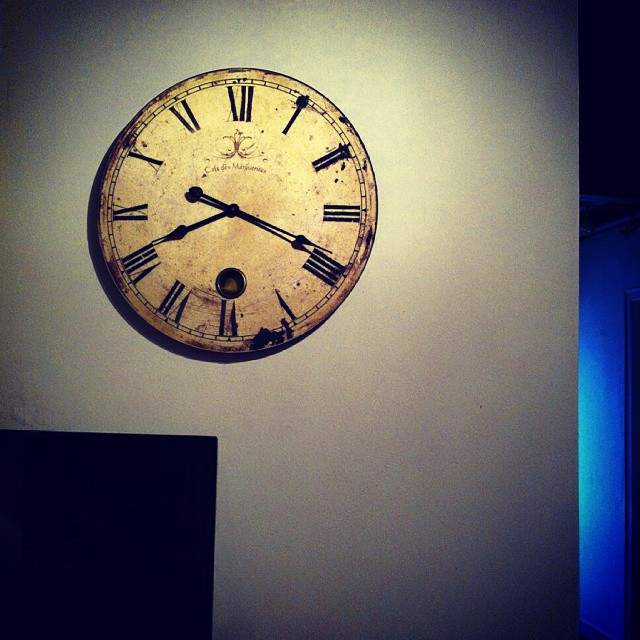The image presents a low-lit and slightly grainy interior setting with a light gray wall in the foreground, contributing to a somewhat washed-out appearance. Dominating the center of this wall is a large, circular, rustic clock that exudes an old and weathered charm, clearly showing its age through a distressed, dirty surface. The clock face is light-colored, adorned with black Roman numerals around its perimeter and a black hand mechanism frozen at 3:41. Characteristically detailed, the clock features a red trademark stamp above the hand mechanism with a floral Fleur de Lis design, accompanied by some cursive script, now too faded to decipher. Below the hand mechanism lies a small, circular cutout with a distressed gold grommet at its base. A shadow from an unseen light source is cast behind the clock, adding depth to the scene. In the bottom left corner of the image, the top right section of a black TV screen is visible. In the far background, the right-hand side of the image reveals an open doorway leading to another room, from which a glowing blue light emanates, casting an ethereal glow into the somber interior.